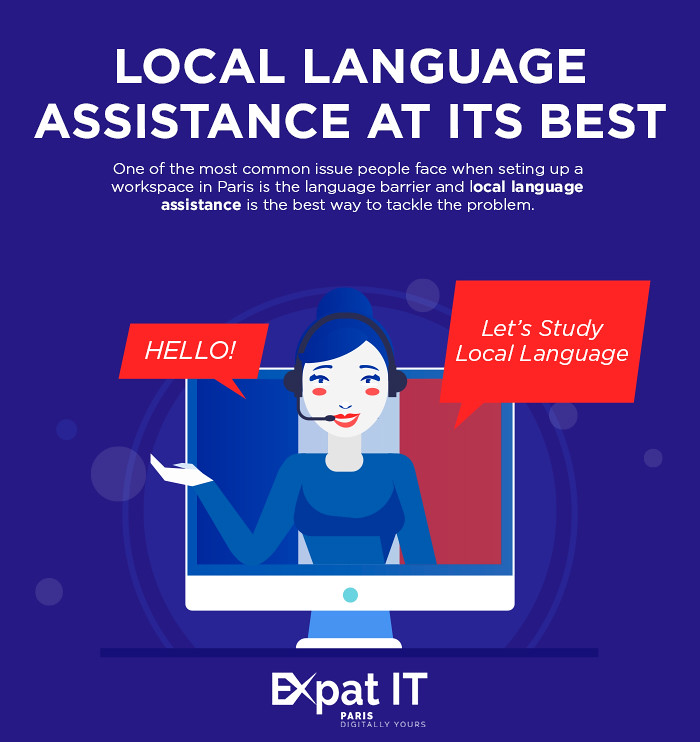The advertisement features a dark blue background and prominently showcases the white text "Local Language Assistance at Its Best" at the top. Directly beneath this headline, smaller white letters explain, "One of the most common issues people face when setting up a workspace in Paris is the language barrier, and local language assistance is the best way to tackle the problem." The central visual of the ad is a clipart-style image of a white computer monitor displaying a cartoon woman. The woman has blue hair styled in a bun and is wearing over-the-ear headphones with an attached microphone. She is partially emerging from the monitor and speaking, with orange speech bubbles on either side of her, saying "Hello" and "Let's study local language." Below this image, in bold white letters, the text reads, "Expat IT Paris, digitally yours," with "IT" prominently highlighted. The background features a light blue hue, complementing the overall design and color scheme.